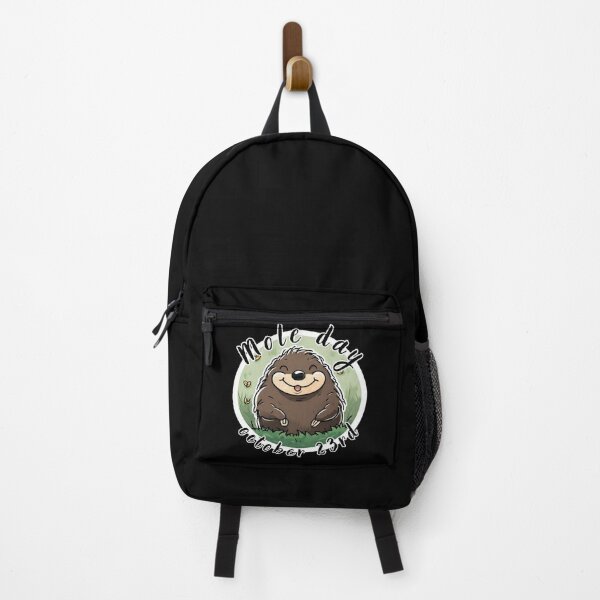The photo captures a black kid's backpack hanging from a wooden hook mounted on a white wall. The focus of the backpack is a circular design situated below the front pouch. This design features a playful illustration of a brown and light brown mole with a black nose, smiling with its tongue out and tiny claws visible. The background of the design includes green grass and light green elements, possibly butterflies, creating a cheerful scene. The text above the mole reads "Mole Day" in black letters with white outlines, while "October 23rd" is printed below the mole. The backpack itself is entirely black, including the zippers, except for a dangling yellow strap.